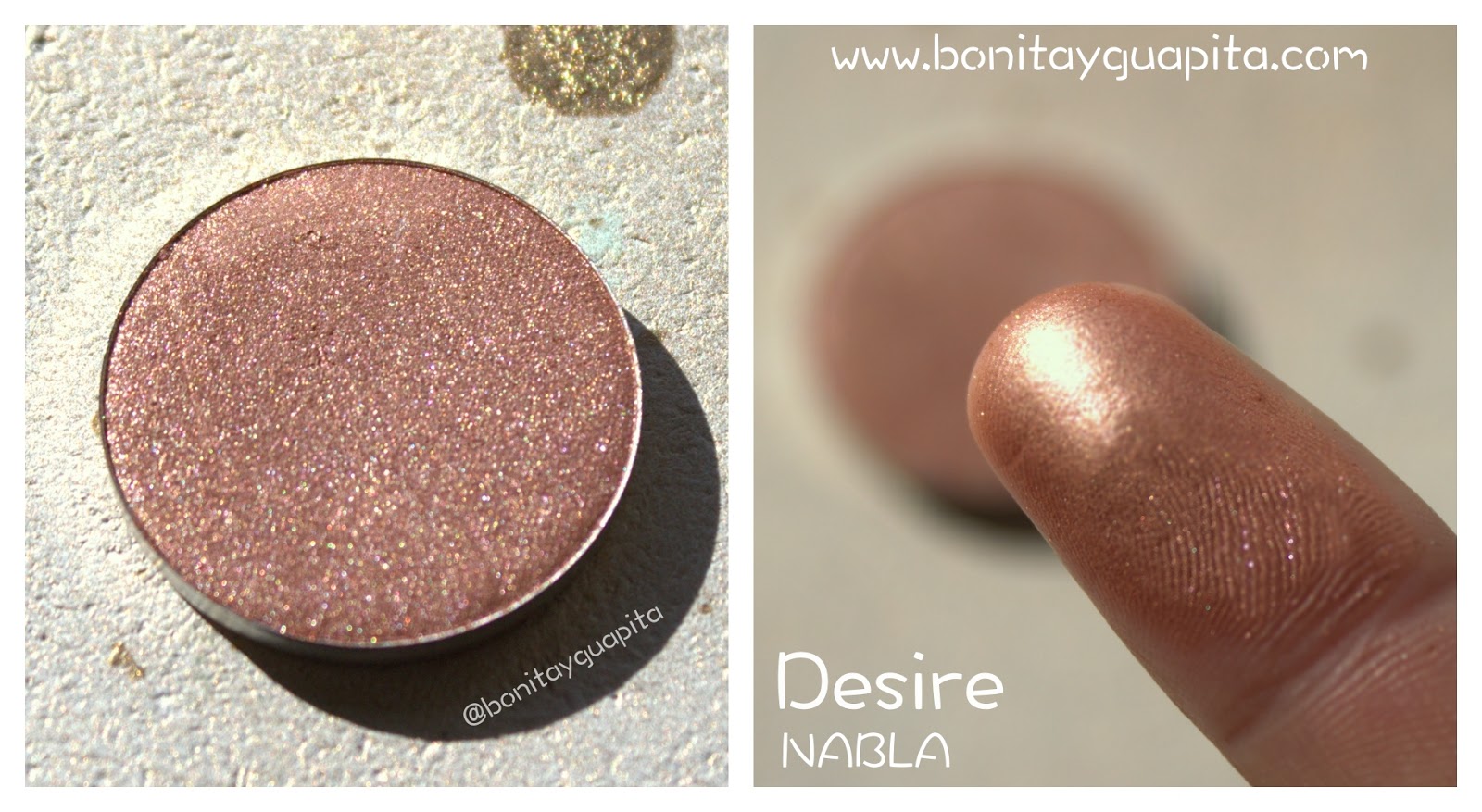The image features a beauty product divided into two side-by-side square photographs, creating a landscape orientation with a white rule separating them. On the left is a close-up of a round tin containing a sparkly cosmetic powder, either foundation or blush, in a peachy golden-pink hue, resting on a textured, pebbly white surface. The cosmetic appears almost coppery, with a small gold spot near the top of the tin. The image includes the social media tag @bonitaguapita. The photograph on the right displays a finger swiped with the same sparkly cosmetic, illustrating its shiny and bright golden-pink color with darker edges. The background here is blurred, giving focus to the fingertip. The top section of the right image features the website URL www.bonitaguapita.com in white letters, while the bottom left corner bears the text Desire Nabla. The combined images exhibit photographic realism and incorporate elements of graphic design and typography.